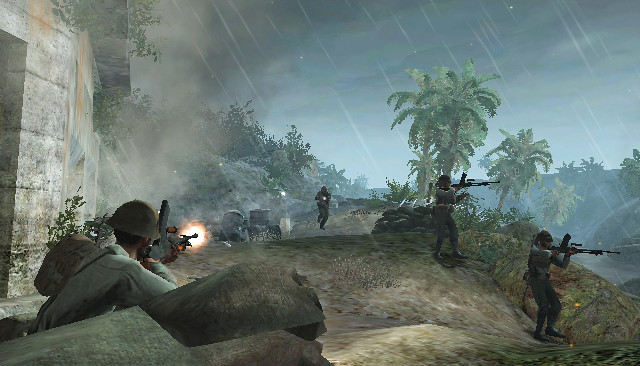This image is a computer-generated screenshot from a war-themed video game, set in a rainy, outdoor jungle environment. The scene features a dark, stormy blue sky with visible dashes of lighter color, representing the rain. The terrain is a dirt surface, somewhat hilly, and dotted with trees, palm trees, and greenery. 

On the left side of the image, there's a stone building and barely visible flag shape, and to its immediate left, a person is partially concealed behind a large rock formation, aiming a gun at another figure running down the hill towards the viewer. The running person is situated on a path that extends from the middle of the screen downwards. To the right of this path, two more military figures are standing and firing their assault rifles towards the right edge of the screen, where the targets are not visible. 

The visual composition places one figure on the immediate left, two centrally, and one in the lower right-hand corner of the image, all engaged in a dynamic, chaotic firefight under the rain-soaked sky.